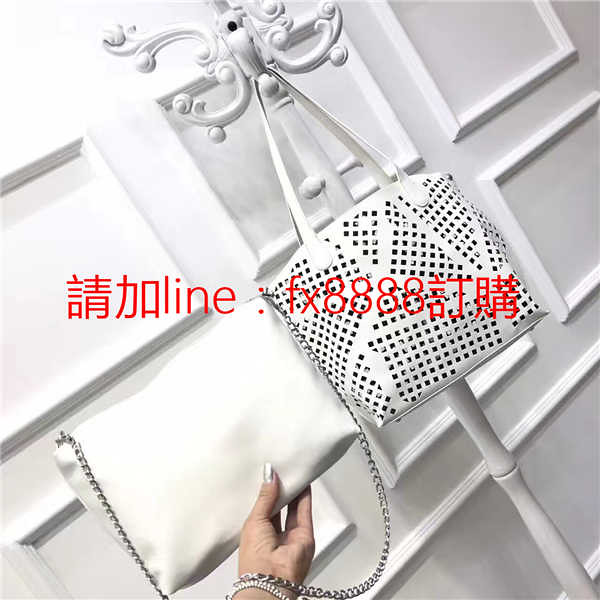This image, likely an advertisement or promotional shot, features a predominantly white backdrop that highlights two elegant handbags. One of the bags is held by a Caucasian female hand adorned with silver nail polish and a silver bracelet, while the other bag hangs from a canted, ornate white coat rack. The held bag is an all-white designer purse with a silver chain shoulder strap, versatile for carrying over the shoulder or arm. The hanging purse also features a white handle and distinctive small square cutouts arranged in triangular and square patterns, creating a see-through mesh effect. Surrounding the bags, the decor includes a white-painted wall with decorative, empty extrusions resembling picture frames, contributing to the image's clean and minimalist aesthetic. Centrally positioned text in Korean accompanies the English character sequence "FX8888," suggesting a foreign or international market context, possibly from a retail platform such as Taobao, AliExpress, or Weibo.